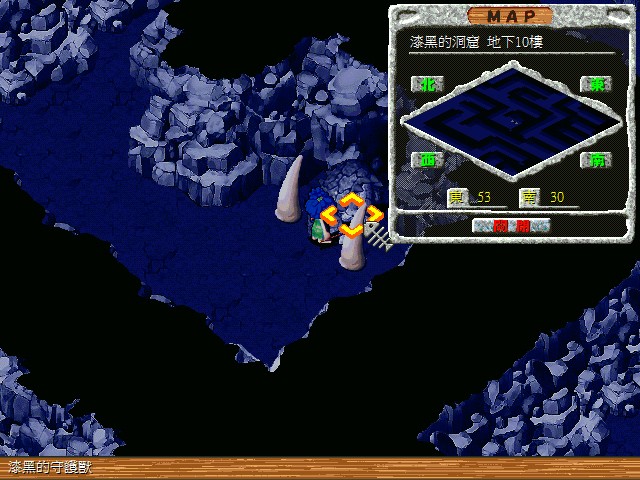This is a highly detailed caption of an image depicting a video game interface:

The image showcases a video game screen with a distinct section across the bottom resembling wood, characterized by a brown hue and visible wood grain patterns. In the bottom left corner, there are characters in either Chinese or Japanese script. The primary screen is dominated by a deep blue background with scattered lighter blue shapes, likely representing rocks, extending from the top left corner downwards and then upward towards the bottom right corner. This pattern creates a dynamic visual pathway across the screen.

In the upper right-hand corner, there is a gray square labeled "map," accompanied by additional Chinese or Japanese characters. This map provides a square-shaped overview of the game area, displaying various characters and numbers indicative of the player's environment. Black sections within this map suggest areas that are inaccessible. Near the bottom corner of the map, two structures resembling teeth or tusks protrude from the ground, alongside a depiction of fish bones.

The game screen features a character standing within a yellow square, further contextualizing the game's scenario and player positioning.